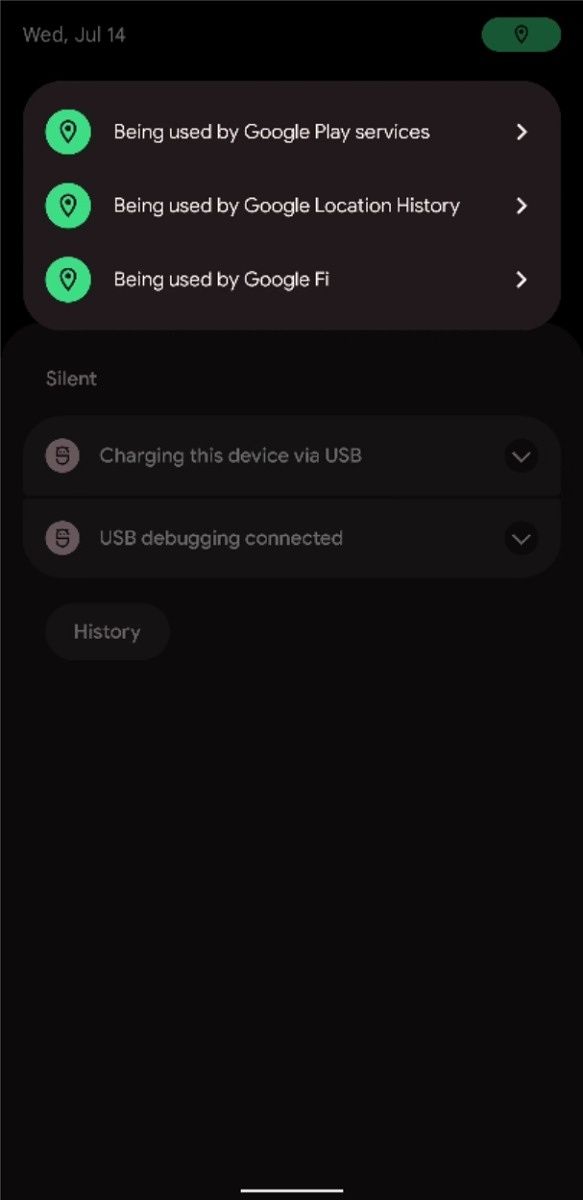This screenshot, captured in mobile landscape mode and utilizing night mode, presents a detailed view of the device's settings interface against a black background. At the top, there's a slightly lighter black box containing various settings, each marked by green circles on the left.

The first setting, “Being used by Google Play Services,” features a green location icon to the left and an arrow pointing right for expansion. Directly below, “Being used by Google Location History” follows the same format with an expandable arrow on the right. The third entry reads “Being used by Google Fi,” also with a right-pointing arrow for detailed options.

Grayed out and labeled at the top left in small white letters is the "Silent" option, indicating a muted notification state. Under this section, two subcategories are present: "Charging this device via USB," with a downward-pointing arrow on the right to show more details, and "USB debugging connected," accompanied by a right-pointing arrow for additional options. At the very bottom left of the interface, a gray button labeled "History" offers access to historical activity records.